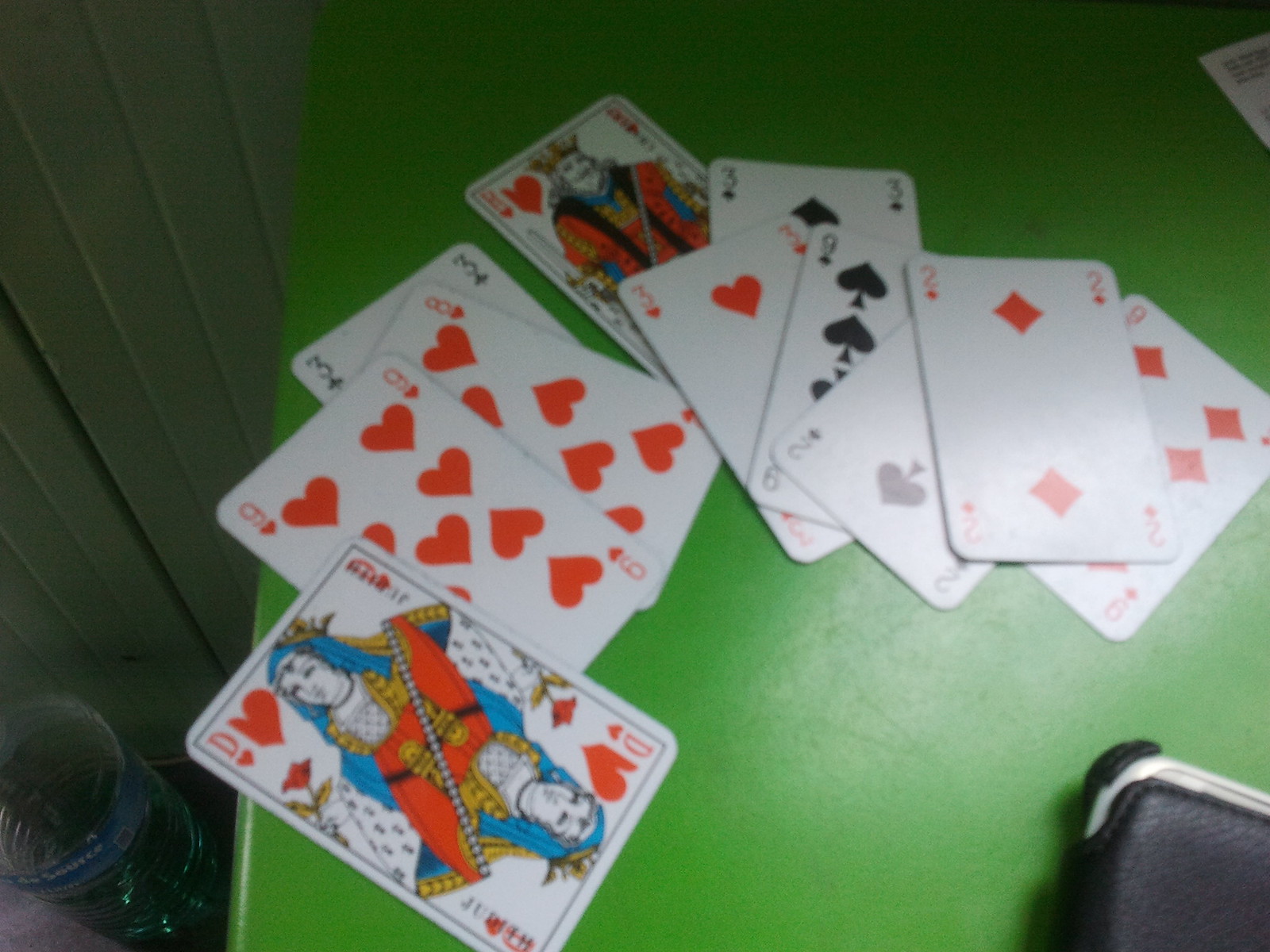This slightly blurry photograph captures an intricate arrangement of playing cards against a detailed backdrop. On the left-hand side, the background features a wall composed of thin vertical white panels which exhibit a greenish-yellow tinge and are cast in shadow. Adjacent to the wall, there is a large, translucent plastic bottle filled with a vivid blue liquid and adorned with a blue label near the top that bears the word "source" in white text. Dominating the right-hand side of the frame is a bright green table. The table is draped in shadow at the top, while a bright, reflective white light accentuates the bottom right corner. Partially visible in the foreground is a leather-like phone case with a small, rounded white object protruding from underneath. The primary focus of the image is a pile of playing cards arranged in an arc extending from the bottom left to the center-right of the frame. Notably, the bottom left features a distinctive card displaying a red Queen of Hearts, illustrated with a woman wearing a blue headdress. Progressing upwards and to the right, the sequence of cards includes the 9 of Hearts, 8 of Hearts, 3 of Clubs, King of Hearts, 3 of Hearts, 3 of Clubs, 9 of Spades, 2 of Spades, 2 of Diamonds, and culminates with the 9 of Diamonds.